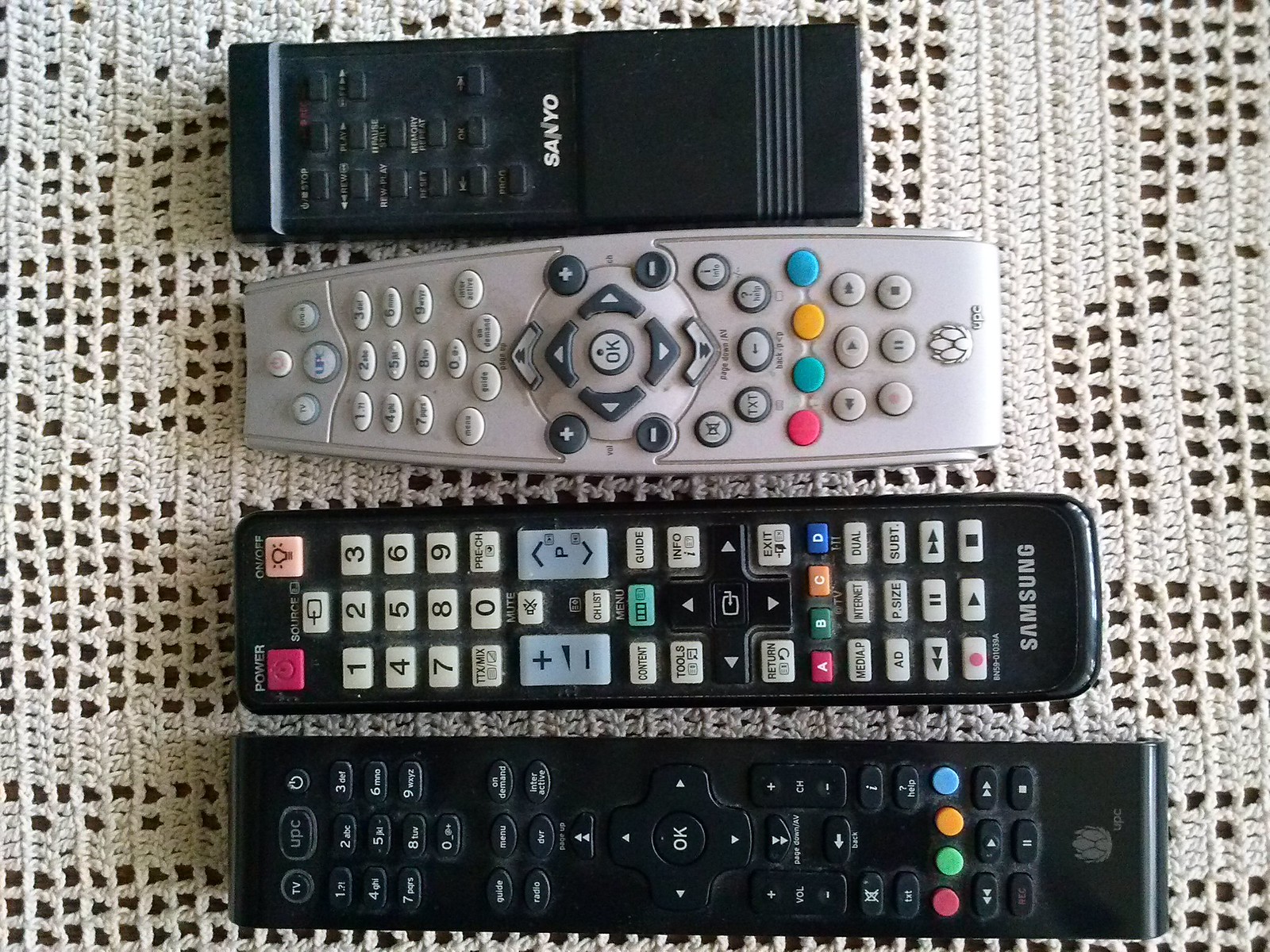The image is a color photograph taken from above, showcasing four TV remote controls neatly arranged in a vertical stack on a delicate off-white crocheted tablecloth. The crocheted pattern of the tablecloth features a series of small, see-through squares, revealing glimpses of a brown wooden surface underneath. Each remote is distinct in color and design, adding variety to the arrangement.

At the top of the stack is a small, simple black remote from Sanyo, featuring about ten buttons. Directly below it is a gray remote with a slightly flared belly, adorned with a central menu button surrounded by directional arrows, volume and channel controls, and a bottom row of colorful buttons in red, green, yellow, and blue.

The third remote is a black Samsung device, recognizable by its square and rectangular buttons, including a notable red power button and a light bulb button on the upper right, possibly for a flashlight function. Finally, the fourth remote, similar in brand to the gray one as indicated by a lotus flower or artichoke logo, is another black remote with black buttons and a distinctive row of colorful circular buttons in red, green, orange, and blue.

This detailed arrangement highlights the mix of button shapes and colors across the remotes, set against the intricate background of the crocheted tablecloth.